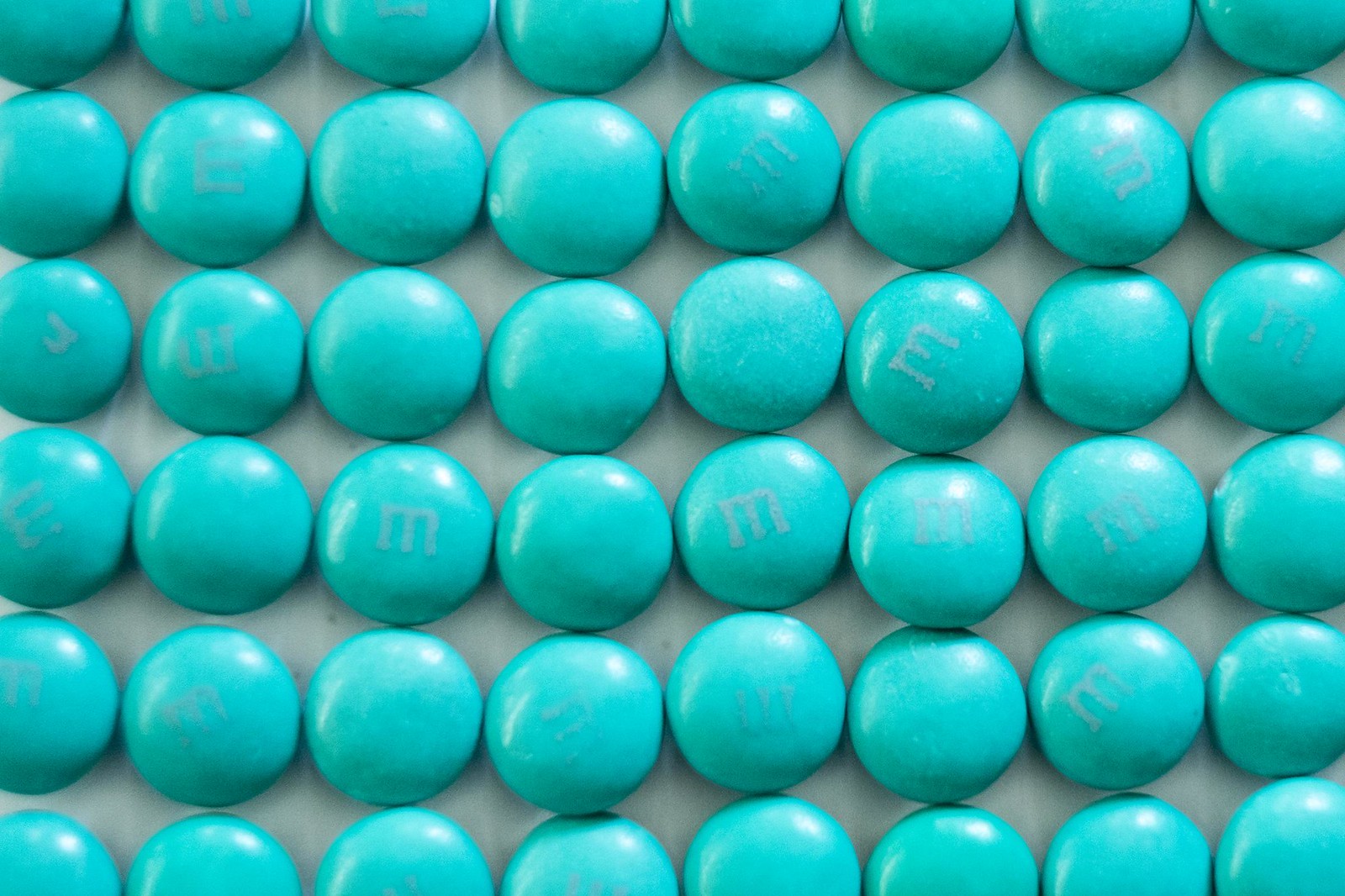This is a detailed close-up photograph of light blue M&M candies arranged in a precise grid pattern. The image features six horizontal rows, each containing eight uniformly shaped and colored M&Ms, making a total of 48 candies. Each candy is round and displays the iconic "M" logo, although in some pieces the "M" might be less visible. The candies have a slight reflective shine, likely from the camera flash or another light source behind the camera. The background surface, visible between the candies, is a light gray or white color, suggesting either cloth or another smooth surface. The overall lighting is bright, highlighting the smooth, painted-like turquoise or aquamarine hue of these M&Ms, creating an artistic and visually neat arrangement.